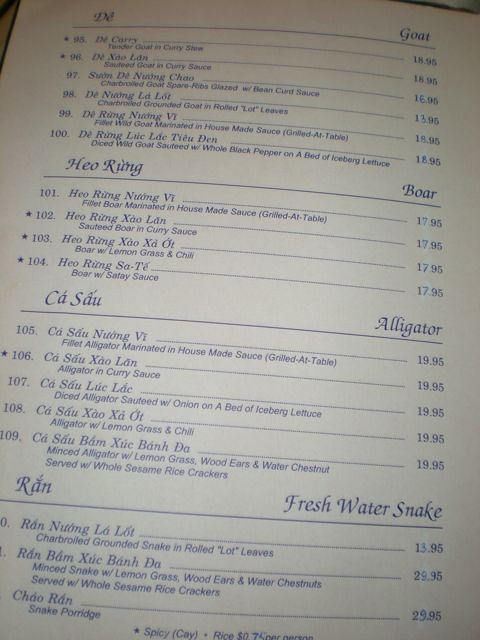A well-worn menu page features both English and a foreign language, showcasing a series of exotic dishes. Each dish's name is first printed in the foreign language, followed by a detailed English description underneath. The menu is printed on white paper with dark gray text, and it is meticulously categorized into four sections: Goat, Boar, Alligator, and Freshwater Snake. Each section includes approximately four to five dishes. On the right side, prices are neatly listed in USD. The photograph captures the menu page in a dimly lit restaurant, which suggests a cozy and intimate dining environment. The page itself appears slightly curved and bent, indicating it has just been turned, hinting at a multi-page menu.